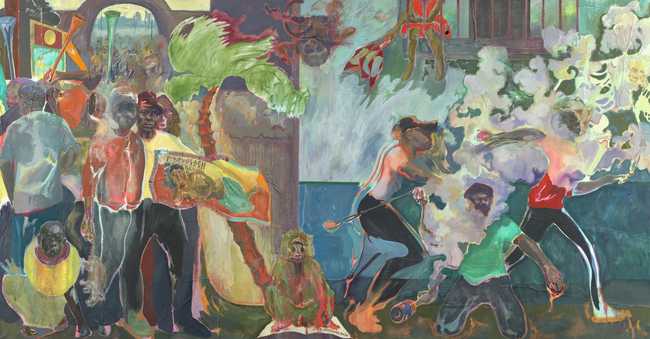The image depicts a vibrant, somewhat abstract, and modernistic painting set in a tropical locale, possibly reminiscent of the Caribbean. Central to the scene is a large palm tree under which diverse groups of dark-skinned people engage in various activities. Some stand, some run, some appear to throw objects, and others give the impression of writing. The background reveals a building with a window featuring bars or a balcony. The people are dressed in colorful attire—yellows, greens, and reds—contrasted by long black pants, and one figure even wears a hat. A notable element is the presence of a monkey, possibly two, positioned at the forefront on the sidewalk. The painting employs a blurred, unclear style, rendering specific features indistinct while enhancing the vivid and dynamic color palette that integrates shades of reds, greens, and blues. Despite its lack of fine detail, the painting powerfully evokes the challenges and everyday life of its subjects, potentially alluding to historical or social narratives. There is no visible signature from the artist, adding to its enigmatic nature.